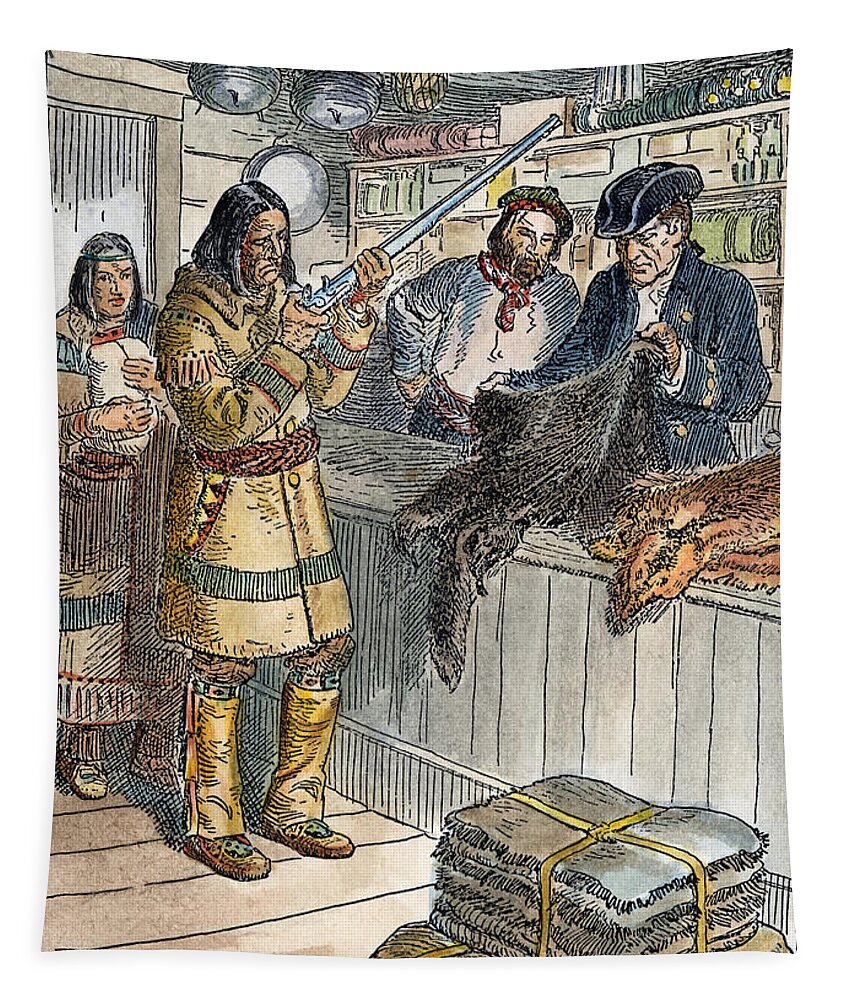This detailed color illustration, reminiscent of the 1700s, portrays a bustling general store scene. In the center, the counter displays various animal pelts, including a black and a brown fur. Behind the counter stand two men: one in a colonial-style jacket and hat, the other donning a hat and scarf, both attentively examining the furs. To the left, two Native American individuals take prominence; the man, holding a long rifle upright, stands in front, while the woman behind him cradles a baby. On the wooden floor in the foreground lies a stack of neatly bundled furs, securely tied with a yellow cord. This vivid depiction captures the essence of historical trade and interaction between cultures in a richly detailed tableau.